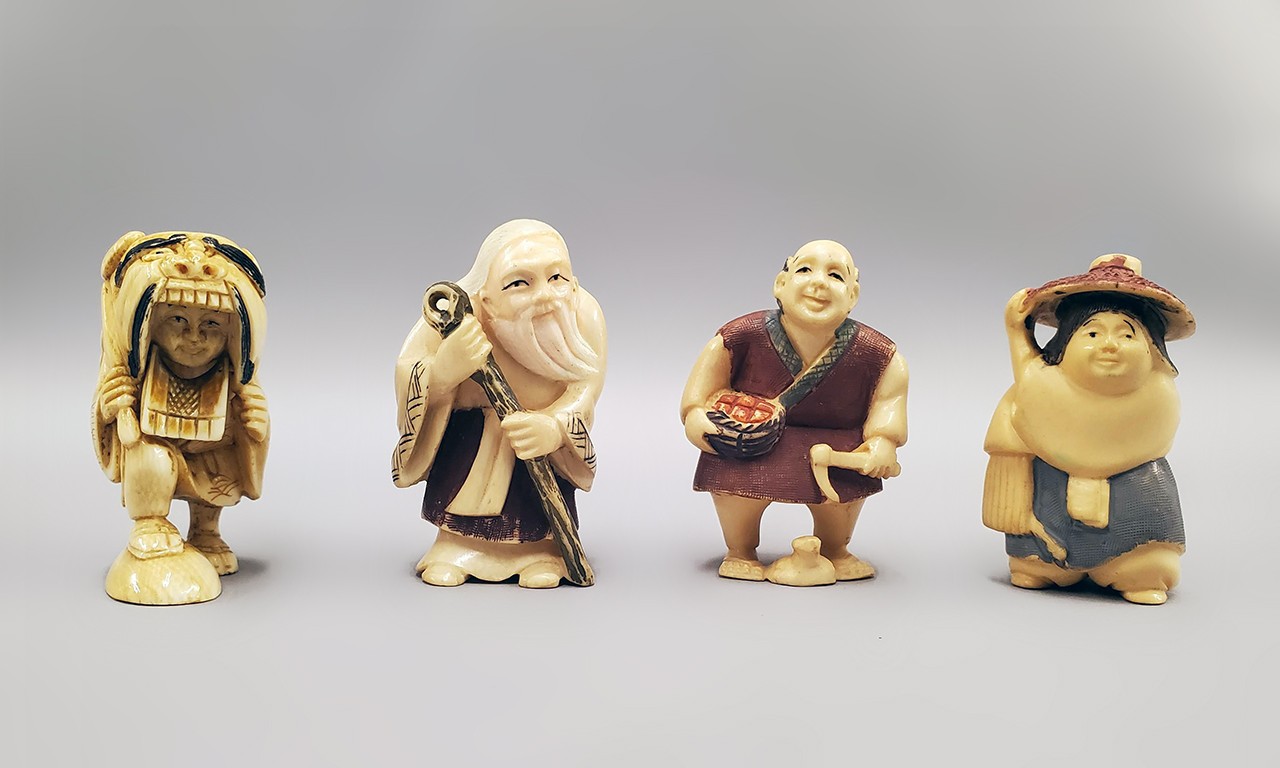The photo features four small, ivory-colored wax figurines arranged in a line against a plain white background, likely taken in a photo box setup. From left to right, the first figure resembles a Native American adorned with a headpiece that drapes down, holding onto it while standing with one foot on a rock. The next figure appears to be an elderly Japanese man with a long white beard, clad in a kimono with wide sleeves and holding a staff in both hands. The third figurine represents another Japanese character, potentially a farmer, holding a basket of apples and a small cutting tool, possibly a scythe. The final figure portrays a chubby Asian man with blue pants, a red hat, and a traditional flat hat, completing the diverse tableau. All figurines exhibit historical or cultural attire, contributing to an old-fashioned, ethnographic aesthetic.